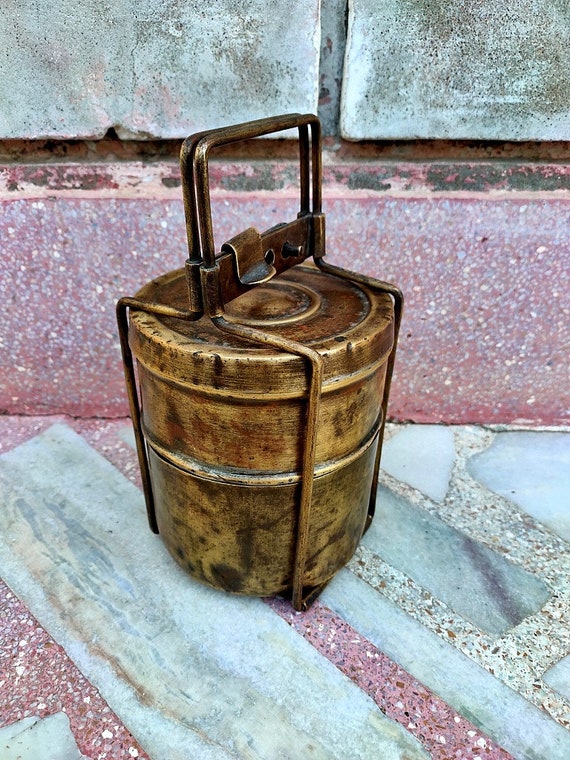The image captures an antique cylindrical canister, reminiscent of an old ice cream maker, with a brushed gold finish adorned with black smudges, giving it a weathered look. The canister features a metal carrying device that clamps around its body with bars ending in two handles, which can be secured together with a small brown leather belt. The canister, appearing both metallic and wooden in parts, displays a mix of light and dark distressed brown colors. It rests on a striking floor of pink, white, and gray marble tiles, with sections of red rock and gray diagonal stones. The background behind the canister continues the pink marble theme, edged by distressed white bricks higher up, adding to the antique ambiance of the scene.